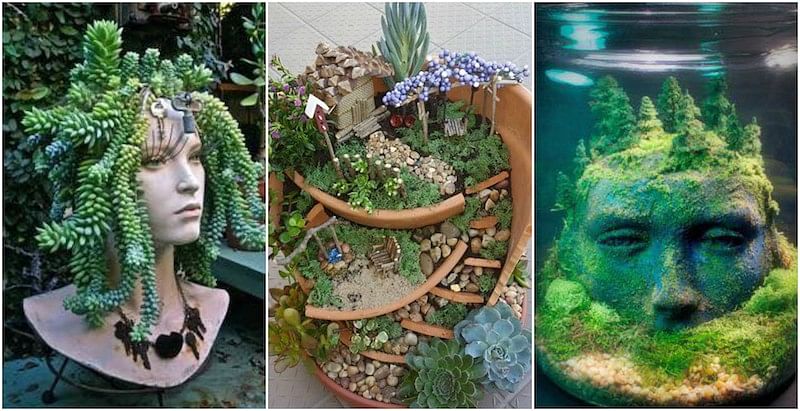The image is divided into three equal-sized panels, each showcasing unique plant displays entwined with artistic elements. On the left, there's a striking sculpture of a woman's head with lush, green plants and cactuses sprouting from it, forming a hair-like appearance. The middle section features a terracotta bowl meticulously crafted into a mock-up garden, complete with a miniature chair, outdoor stove, post box, and bird cage, all enveloped in greenery. The right panel displays another head submerged in water, its surface adorned with green moss and plants, evoking an ethereal, Aquarius-like theme. The combination of these elements gives the image a surreal and captivating nature-inspired aesthetic.